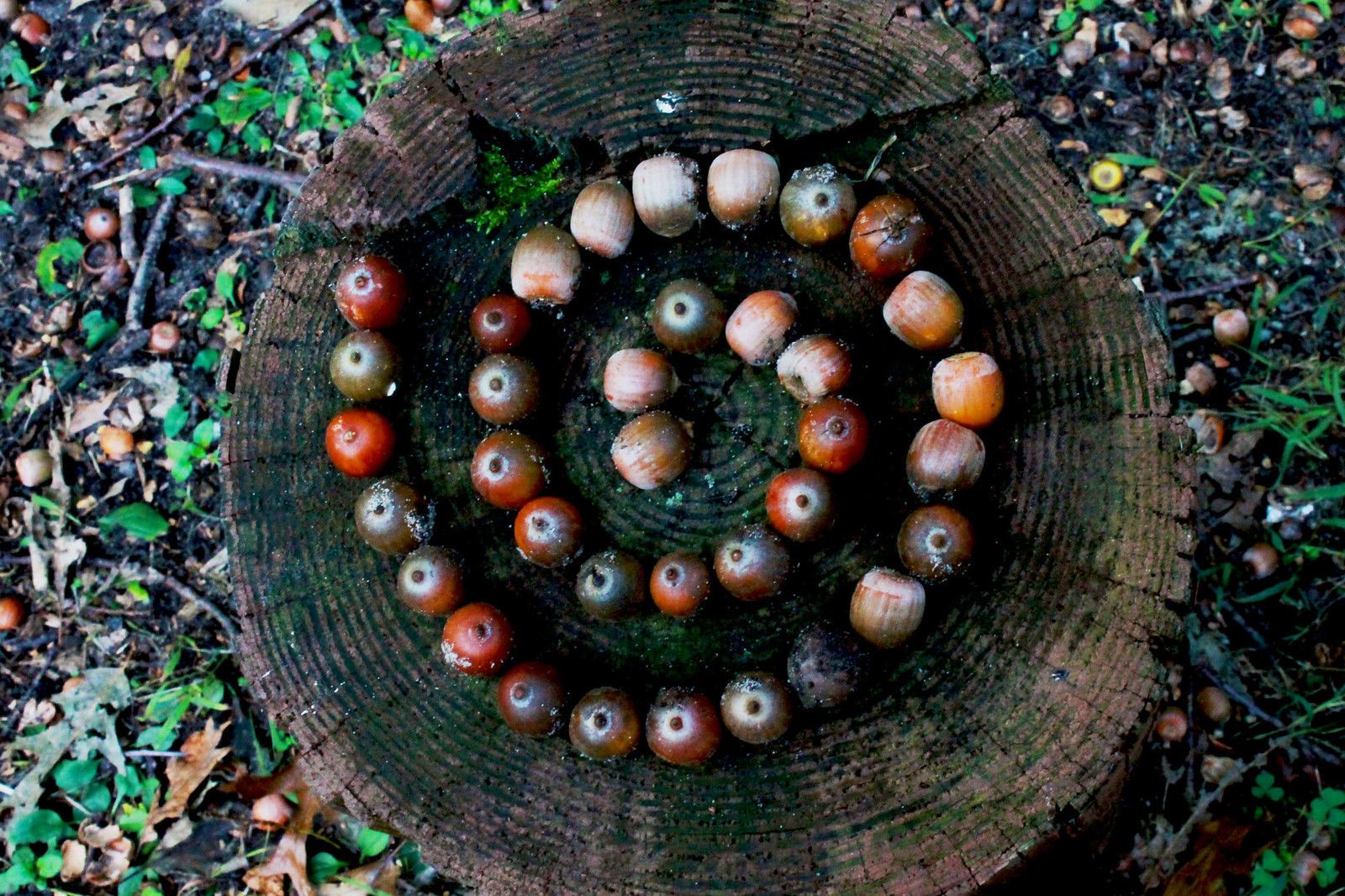The photograph captures an overhead view of an old, cut tree stump in a forested area, revealing the dark, decaying rings and inner trunk. Arranged meticulously on the muddy, partially moss-covered surface of the stump is a spiral formation of small, circular fruits, which could be mistaken for acorns but resemble tomatoes with vertical striations and a bloom on their skin. These fruits vary in color, ranging from shades of pinkish-red and deep red to green and beige, each with a little stem on top. The surrounding ground is damp and scattered with additional fruits, broken tree limbs, brown leaves, green grass, and twigs, contributing to the earthy and natural ambiance of the scene.